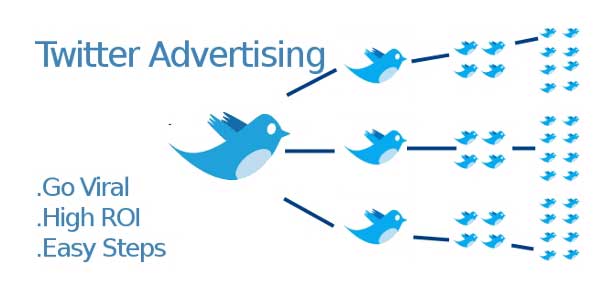This screenshot showcases a website focused on Twitter advertising. The header features the text "Twitter Advertising" with "Twitter" in uppercase and "Advertising" in a mix of uppercase and lowercase letters, all set in a blue font. Below the header is Twitter's iconic blue bird logo, prominently displayed. The medium-sized bird is in the center and features three extending lines positioned at 1 o'clock, 3 o'clock, and 5 o'clock. Each of these lines branches out into additional lines and birds: 

- The line at the 1 o'clock position leads to one bird, which then splits into four more birds, further branching into eight additional birds.
- Similarly, the line at the 3 o'clock position also connects to a single bird that extends into four more birds, and finally, eight birds.
- The line positioned at 5 o'clock follows the same branching pattern as the previous lines.

To the left of the blue bird graphic are three bullet points: "Go Viral," "High ROI," and "Easy Steps," all written in light blue text. The entire design is set against a crisp white background, creating a clean and modern aesthetic.